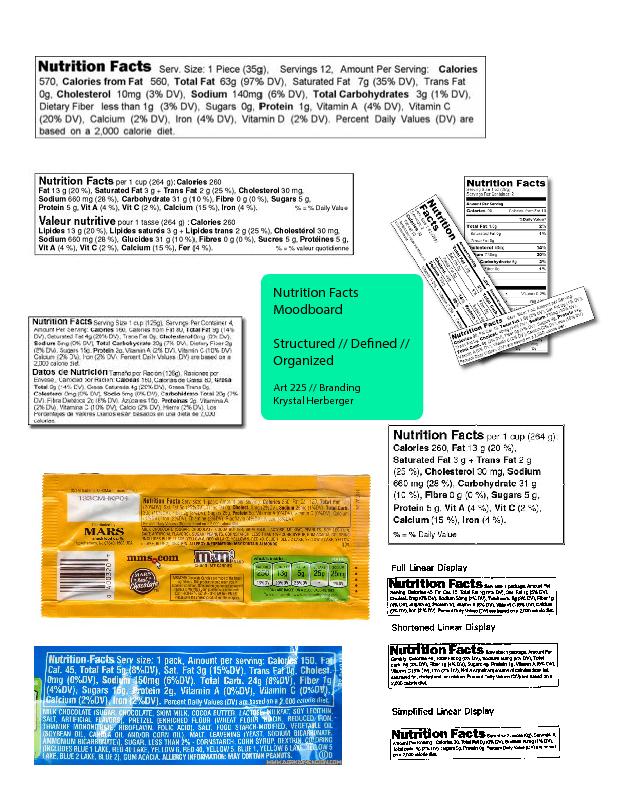This image showcases a meticulously crafted project titled "Attrition Facts Mood Board," conceptualized and assembled by Crystal Herberger as part of her R-225 Branding coursework. Central to the mood board is a prominently displayed title, inscribed in bold black letters against a striking green square, declaring "Attrition Facts Mood Board: Structured, Defined, Organized."

At the apex of the board, we find a detailed Nutrition Facts label extracted from an unspecified food product, isolated within its own square frame. Beneath this, a slightly smaller but equally isolated Nutrition Facts box continues the theme, its textual content too diminutive to assign to a particular food item. Progressing downward, another Nutrition Facts label appears, its minute print further emphasizing the board's intricate examination of such labels.

A notable highlight is an empty M&M's peanut wrapper strategically positioned to reveal only the back label, serving as a tangible connection to real-world packaging. Adjacent to this, a similar yet indeterminate food wrapper, possibly candy, is presented with a distinct glued appearance.

Adding complexity to the arrangement, a small collage emerges, featuring overlapping Nutrition Facts labels of varied sizes: one notably small, juxtaposed with two of moderate proportions. This layered composition underscores the diversity of food labeling.

Concluding the visual narrative, the bottom section includes another solitary Nutrition Facts label encased within a box, accompanied by three additional photocopies. These copies are seemingly intended to match corresponding food products, completing the mood board's diligent exploration of food package nutrition information.

Crystal Herberger's work encapsulates a thorough and organized presentation of Nutrition Facts, embodying the essence of structured branding analysis.